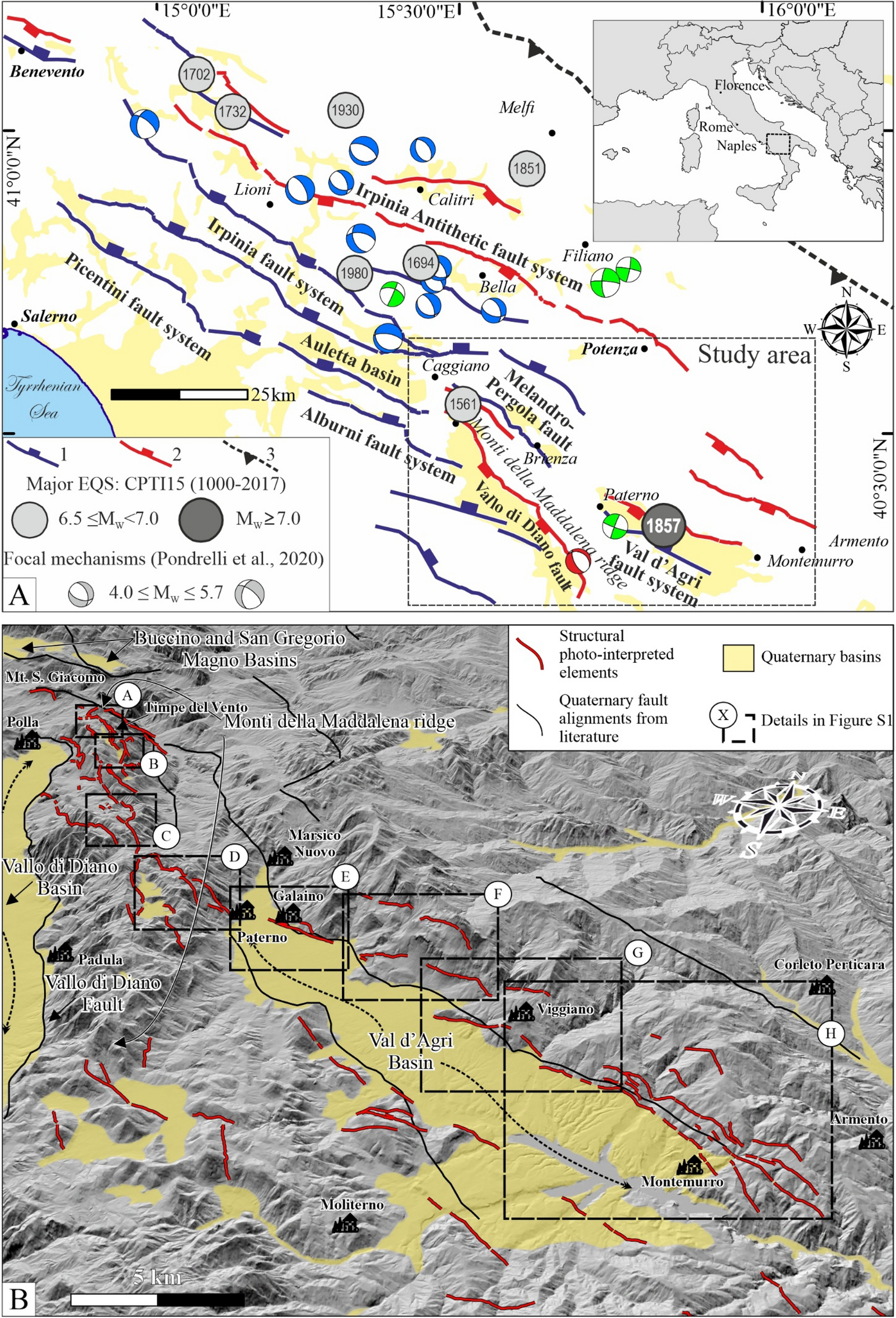This color illustration features a detailed study map of the Urpinia antithetic fault system, divided into two main sections. The upper section has a white background and is densely marked with numerous black and red lines representing various fault systems and fault lines, along with blue and white circular symbols. A key in the top right corner deciphers these elements: red lines indicate "Structural Photointerpreted Elements," thin black lines represent "Quaternary Fault Alignments from Literature," and yellow signifies "Quaternary Basins." An inset map of Italy, highlighting Florence, Rome, and Naples, is positioned in the upper part, with a small box pinpointing the study area near Naples. The lower section showcases a more realistic topographical map with a gray backdrop, emphasizing the raised details of the fault lines and other terrain features. A compass is located on the right-hand side, helping to orient the viewer.